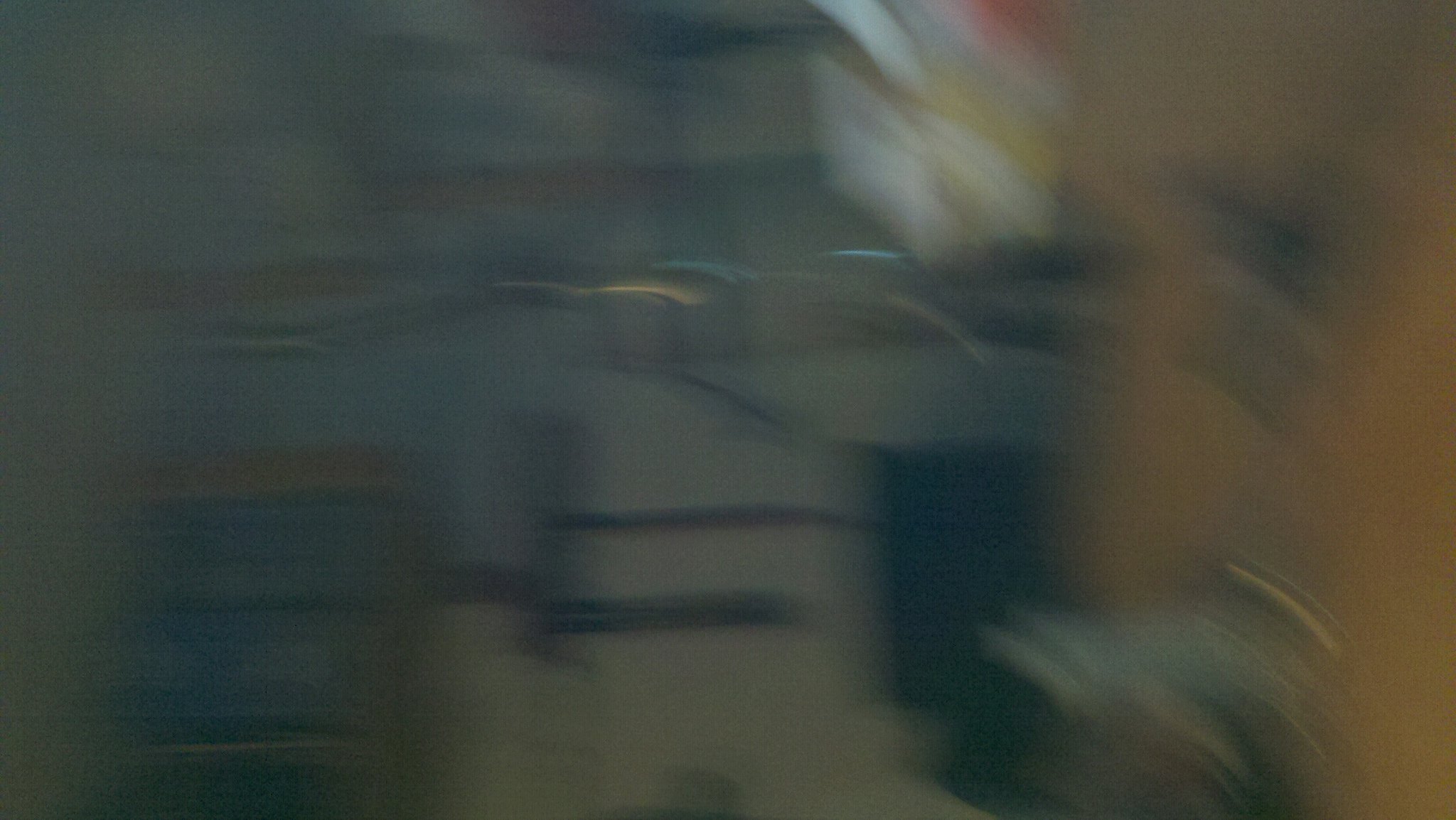This image, taken indoors, is notably blurry and appears to be captured under low light conditions, making it difficult to discern specific objects. Predominantly showcasing hues of gold and brown, the image suggests the presence of furniture common to either a residence or a business environment. A focal point might be a short, brown wooden bookshelf, potentially holding blue-bound books, although this is speculative due to the blurriness. Towards the right side of the image, the scene transitions into solid brown tones interspersed with streaks of gray, accompanied by indistinct black lines and shapes. Notable amid the blur, near the upper center, is a white patch accented with traces of yellow and red. No clear light source is visible, contributing to the overall ambiguous and obscured quality of the photograph.